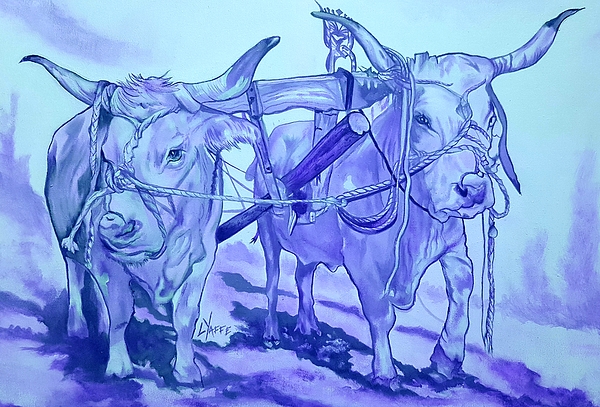This detailed drawing, dominated by various shades of purple, depicts two small, miniature oxen walking through a path, linked together by a complex harness contraption. The entire image is heavily shaded in purple, ranging from dark to light tones, providing a mellow ambiance. The oxen, which have short legs and long, dark-tipped horns, appear to be rather thin. They are tethered together by a wooden yoke that rests heavily on their backs and is tied around their ears. Additionally, they have ropes around their noses, connecting them as they walk. One ox looks straight ahead while the other glances slightly to the right, and the front left leg of one is raised, suggesting they are mid-step. Shadows in dark purple accentuate the overall somber feel of the scene against a predominantly white background. The attention to detail in the shading enhances the appearance and emotion of the piece, making the oxen look noticeably unhappy.